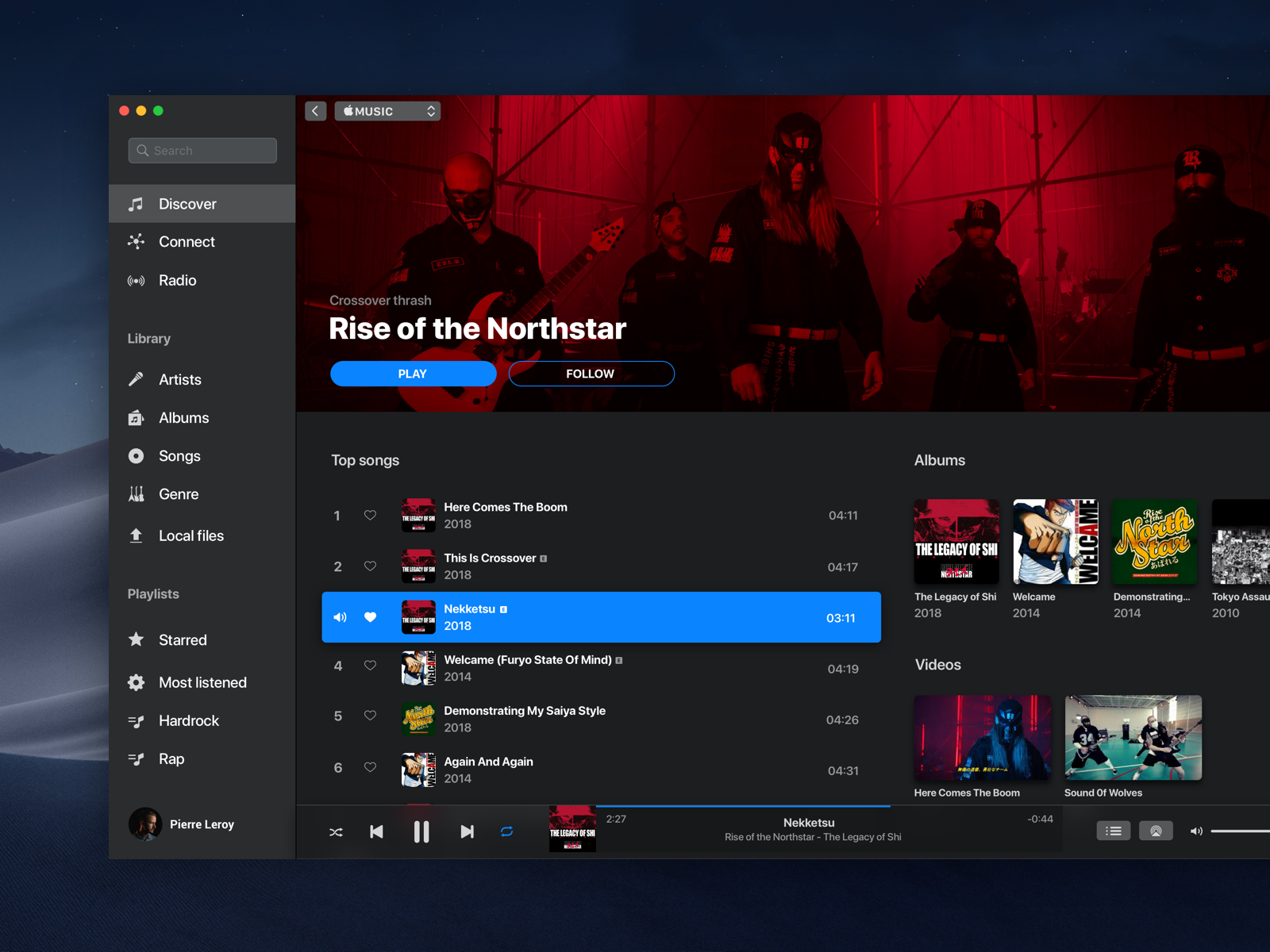The image depicts a user interface of a music streaming application. On the left side, a vertical grey sidebar features a menu listing the following options from top to bottom: Discover, Connect, Radio, Artist, Album, Song, Genre, Local Files, Starred, Most Listened, Hard Rock, and Rap. Below these options is a profile section showing a small profile picture of an individual named Pierre Leroy.

Dominating the top of the main area, there is a large red and black banner image of a band comprising five members, one of whom is holding a guitar. The banner displays the band's name, "Rise of the North Star." Below the banner, two buttons are present: a "Play" button and a "Follow" button.

Beneath the banner, another grey section titled "Top Songs" is displayed. It lists the top five songs of the band with the following information:

1. "Here Comes The Boom," released in 2018.
2. "This Is Crossover," released in 2018.
3. (This spot is unreadable.) 
4. "Welcome, Furo State of Mind," released in 2014.
5. "Demonstrating My Sega Style," released in 2018.